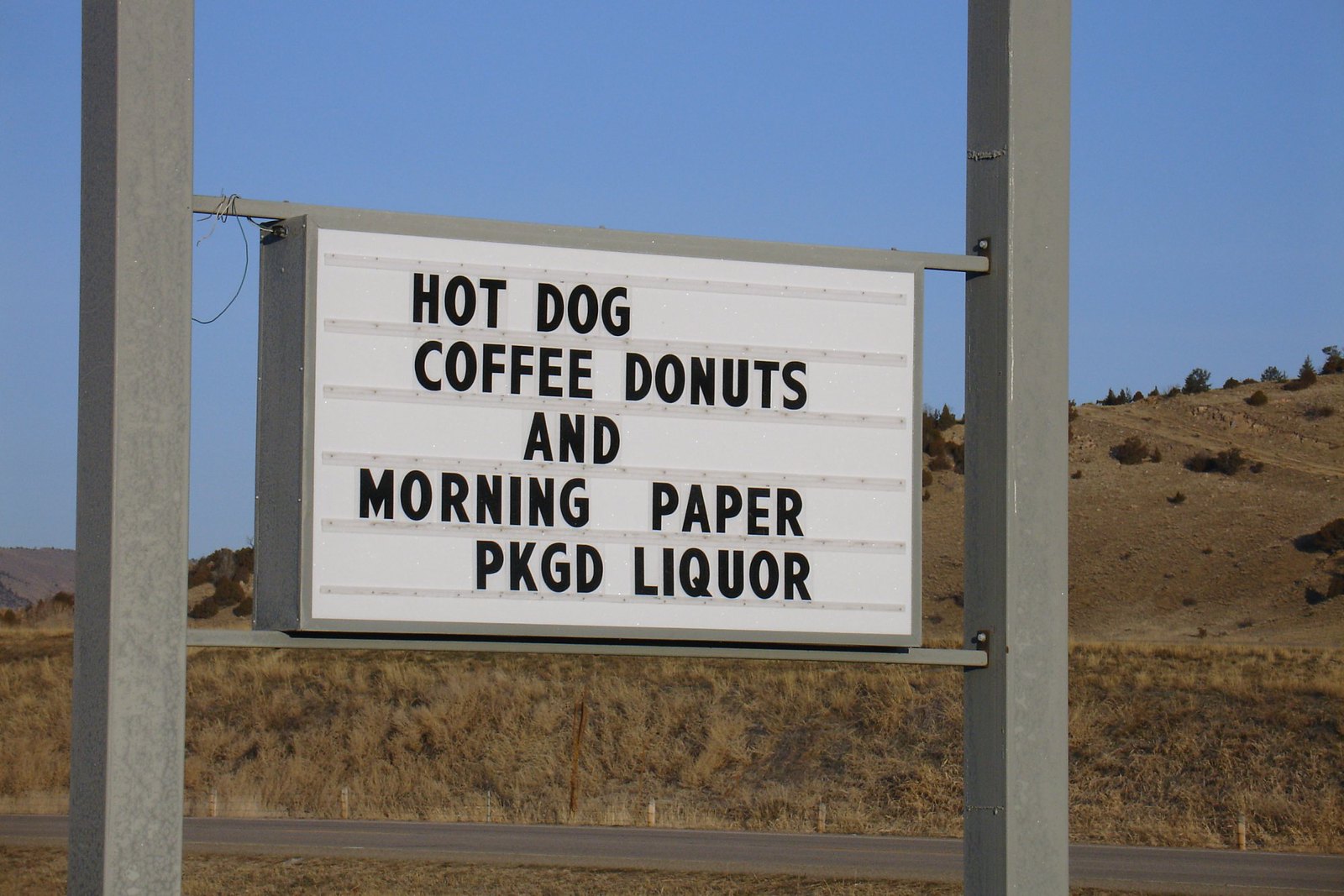A modern photograph depicts a desolate, arid landscape, suggesting desert surroundings. Dominating the image is a prominent white sign with a changeable letter system, set against a stark, blue, cloudless sky. This sign, supported by two sleek, metallic silver pillars, details offerings from a nearby convenience store: "HOT DOG" on the top row, "COFFEE, DONUTS" on the second row, "AND" on the third, "MORNING PAPER" on the fourth, and "PKGD LIQUOR" on the bottom line, all in straight black capital letters. The scene is framed by a barren, brownish terrain with minimal vegetation consisting of dark, withered bushes and short, bare trees. Gentle hills, almost mountain-like, rise in the background, dotted with dead grass and sand, further emphasizing the sense of isolation. A two-lane asphalt road runs alongside the sign, reinforcing the imagery of a remote truck stop or gas station out in the middle of nowhere.